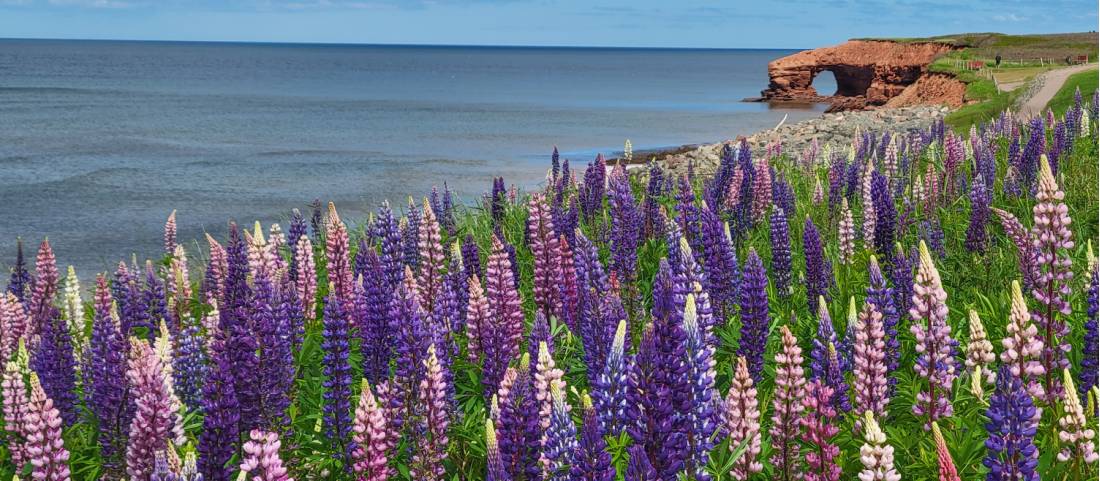A vibrant, color photograph captures a breathtaking partial angle view of a hillside field of lavender, overlooking a calm, medium blue ocean. The foreground is a riot of texture and color with tall blooms in various shades of deep purple and light pink, some featuring delicate whitish tips, all nestled amongst lush, green grass. To the right, a small, brown dirt road winds along the hillside, lined with silver-gray guardrails to prevent cars from plunging into the sea. This one-lane road is partly concealed by the topography, revealing itself only on the right where the land dips lower. Also to the right, a dramatic rocky formation juts out into the ocean, adorned with a natural circular hole that frames a view of the tranquil water beyond. In the distance, a person strolls along the shoreline, adding a subtle human presence to this serene, coastal landscape. The photograph is wider than it is tall, emphasizing the expansive beauty of this scene under a clear, cloudless blue sky.